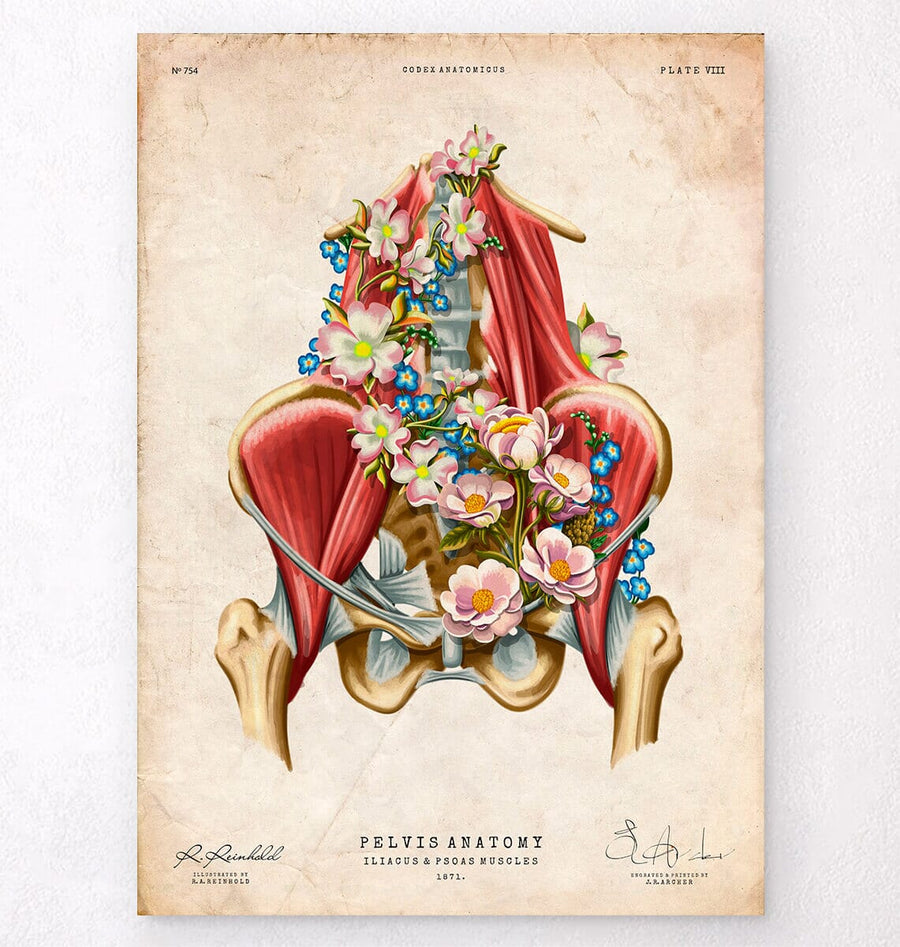The image is a colorful, detailed rendering reminiscent of a page from an anatomical book, showcasing the pelvis anatomy of a human. The background of the page is beige and weathered, indicating its age. Dominating the center is a sizable illustration of the pelvis, prominently colored in red to highlight the bones and muscles. A unique artistic addition is a floral arrangement that weaves through the pelvis, where pink flowers with yellow and orange centers, and smaller blue flowers, are interspersed throughout the bone structure, extending from the spine down to the leg sockets. 

At the top of the page, the labels read "Number 754" on the left, "Codex Anatomycus" in the center, and "Plate VIII" in Roman numerals on the right. The bottom of the image contains the title "Pelvis Anatomy," followed by "Iliacus and Psoas Muscles," and is dated "1871." The bottom corners of the page display cursive signatures in blue ink, which are difficult to decipher. This blend of anatomical detail and artistic flourish creates a visually captivating and informative piece.